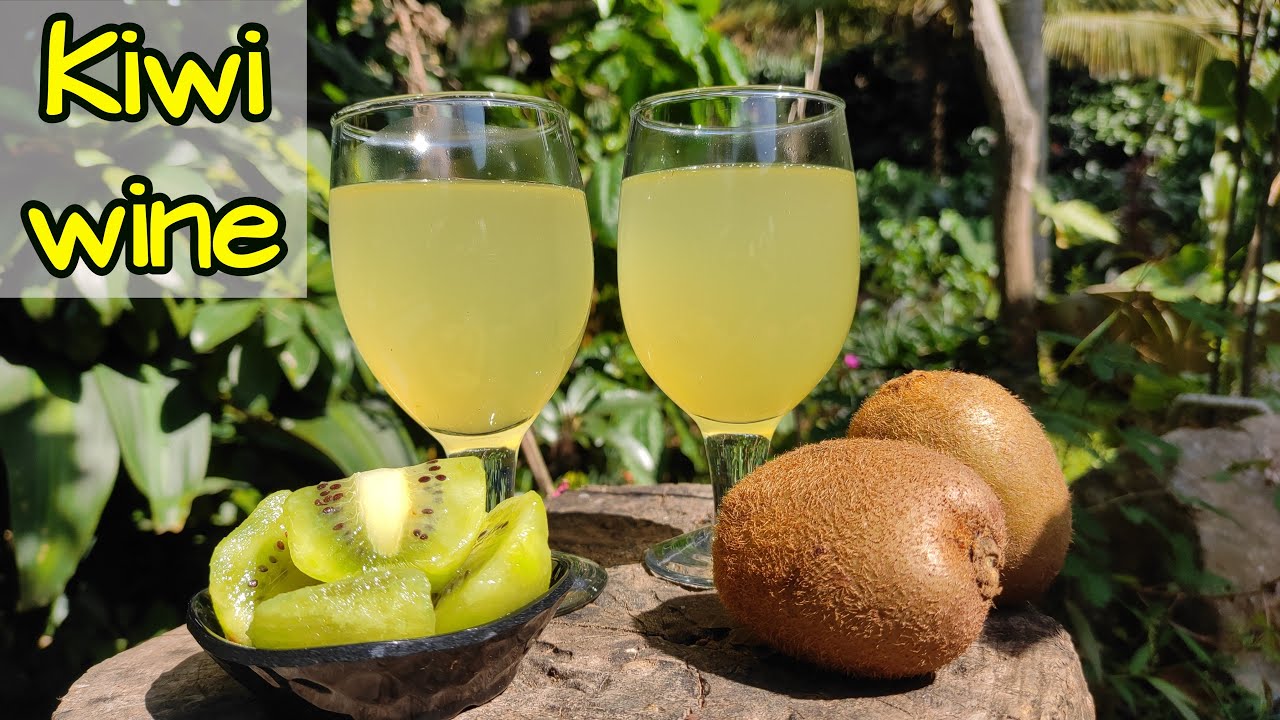This outdoor photographic image, taken during the daytime, showcases two elegant wine glasses filled almost to the brim with a light yellowish-green, semi-transparent liquid presumed to be kiwi wine. These glasses rest on a rustic wooden stump, evoking a natural and serene setting. To the right of the glasses are two whole kiwis with their tan, fuzzy skins intact, while to the left, a black bowl filled with neatly sliced, vibrant green kiwi pieces, complete with black seeds, adds a pop of color and texture. The background features slightly out-of-focus green bushes and trees, contributing to the tranquil ambiance. In the top left corner, the words "kiwi wine" are prominently displayed in yellow font against a transparent gray overlay. The interplay of colors and natural elements beautifully contrasts with the organic setup. Lastly, a solid black block in the bottom right corner balances the image composition.